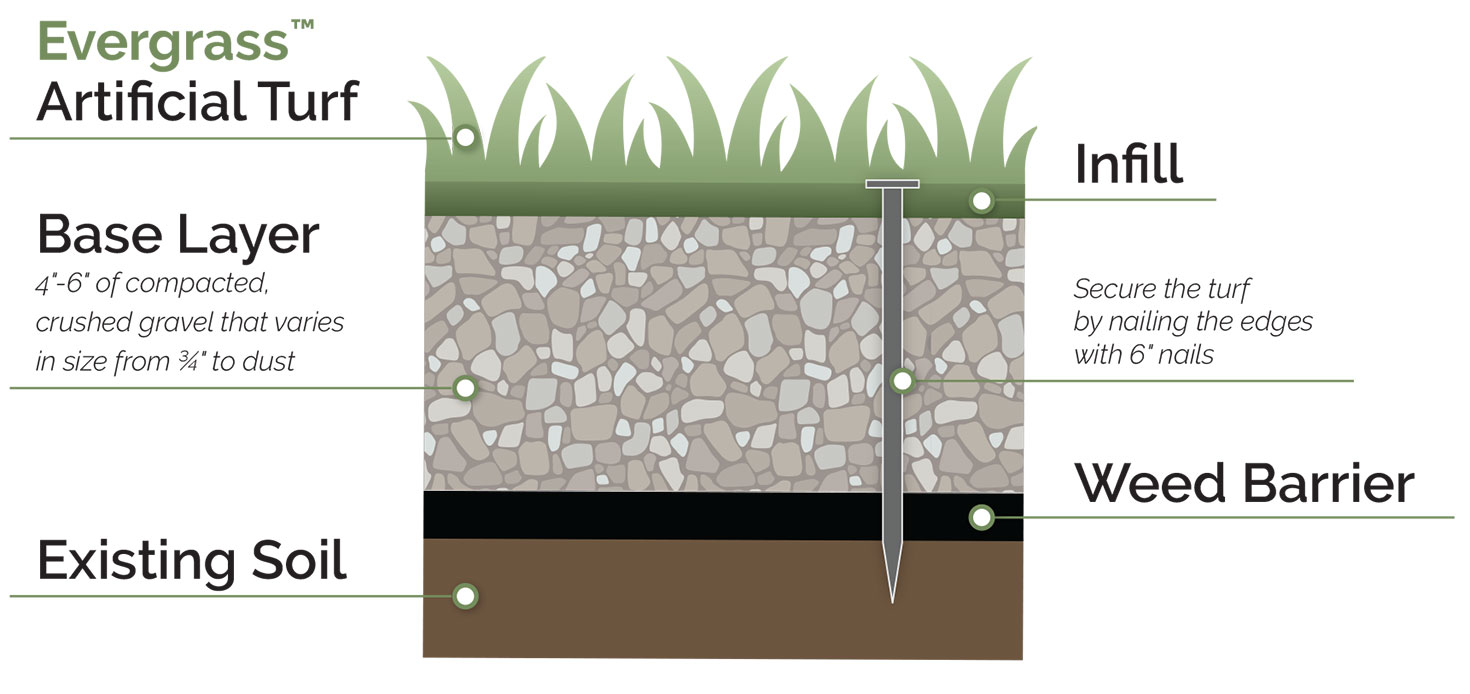The image is a detailed infographic about Evergrass artificial turf, showcasing a layered diagram of its installation process. Positioned prominently, the top of the infographic features the word "Evergrass" in green and "artificial turf" in black. The diagram illustrates the various components from bottom to top: 

1. **Existing Soil**: Depicted at the bottom in brown, representing the natural ground.
2. **Weed Barrier**: A black protective layer placed above the soil to prevent weed growth.
3. **Base Layer**: Consisting of 4 to 6 inches of compacted crushed gravel, varying in size from three-quarters of an inch to dust, represented in gray.
4. **Infill**: Pictured as part of the base that supports the turf.
5. **Evergrass Artificial Turf**: The topmost green layer, representing the synthetic grass surface.

Additionally, the infographic highlights the importance of securing the turf with six-inch nails along the edges, with one nail explicitly illustrated mid-diagram. The overall visual and textual elements are clearly arranged, providing a comprehensive guide for achieving optimal results with Evergrass artificial turf, emphasizing the quality and detailed process of installation.